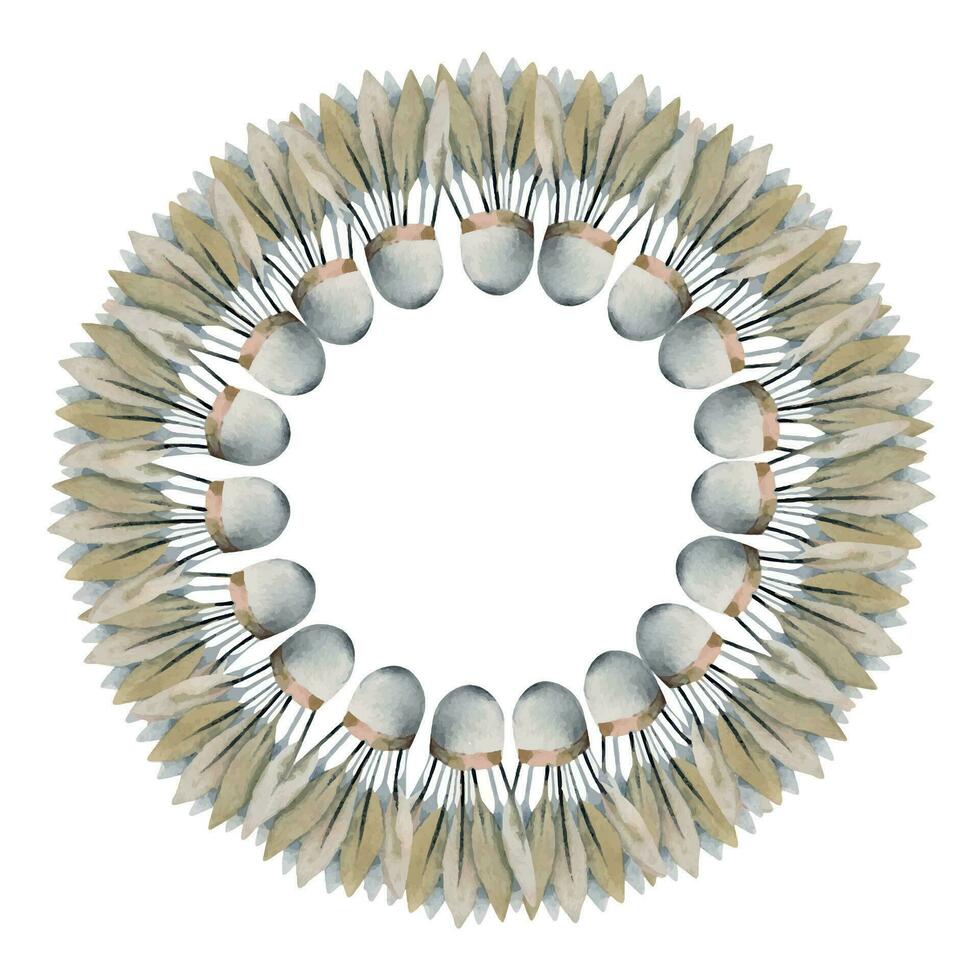The image resembles a detailed color pencil drawing, possibly incorporating watercolor elements. It features a meticulously arranged circular pattern of approximately 19 to 20 badminton shuttlecocks, commonly known as birdies. These shuttlecocks are composed of natural, leaf-like feathers that form the outer edge of the wreath-like shape, giving the overall appearance of a dandelion flower or a decorative door wreath. The feathers showcase a palette of black, white, tan, cream, and shades of reddish brown, with some hints of gray and gold. The central rubber tips of the shuttlecocks are directed inward, creating an open white space in the middle of the circle. The background of the image is white, heightening the intricate and delicate arrangement of the shuttlecocks.